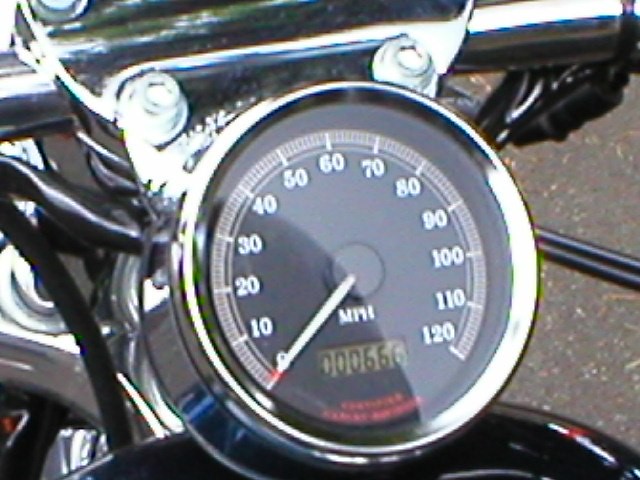A slightly blurry image captures the speedometer of a vintage or retro-styled motorcycle, reminiscent of a Harley Davidson. The speedometer, encased in a shiny, chrome-like frame, reads zero, indicating that the motorcycle is stationary. The odometer shows that the bike has traveled 666 miles. Large screws securing the speedometer to the bike's frame are visible, adding to the rugged aesthetic. The pavement below is partially visible through the bike's frame. The reflective cover of the speedometer gives a faint glimpse of the photographer in its surface.